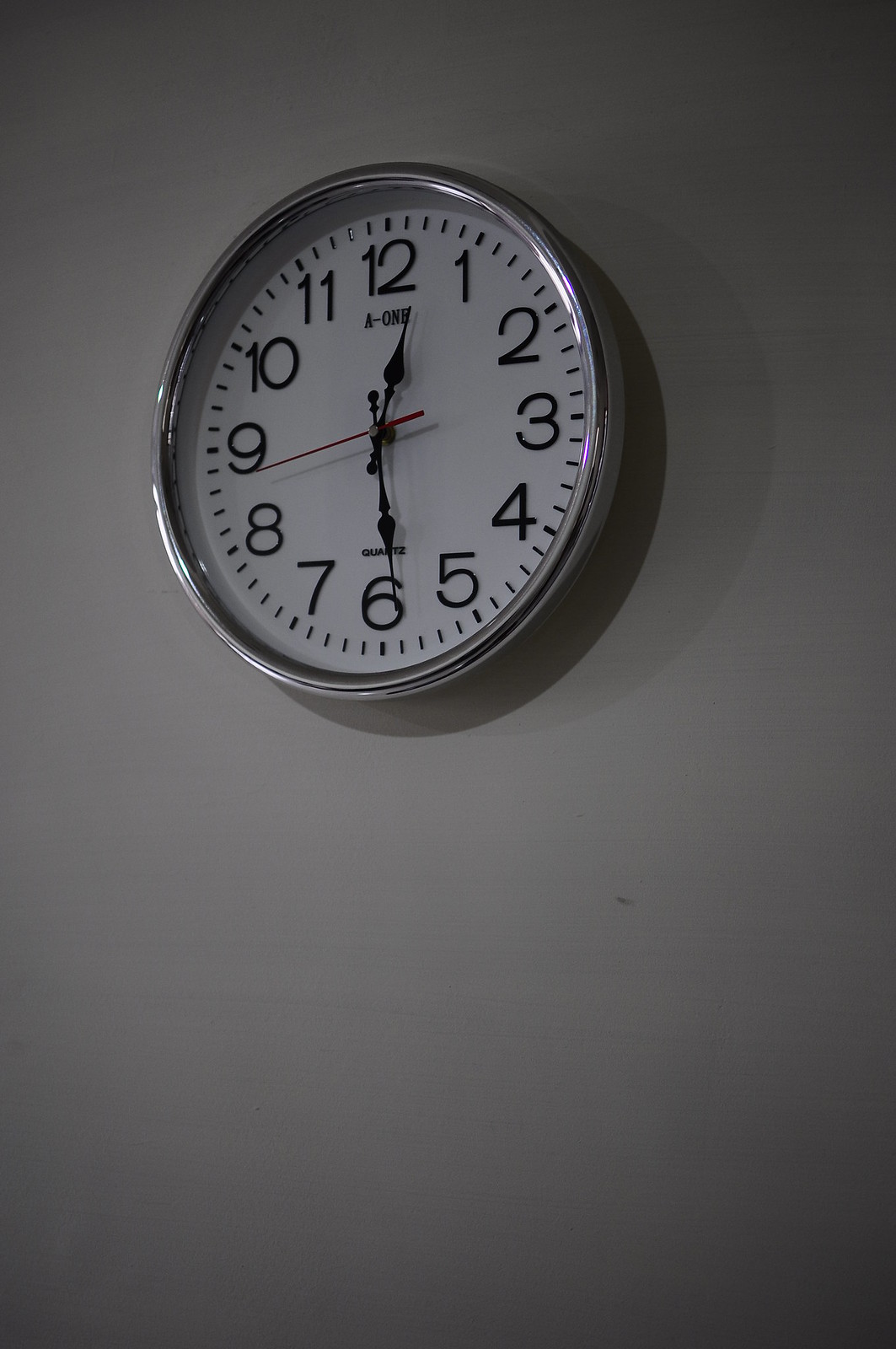The image depicts a wall clock mounted on a pale gray wall. The clock is round with a shiny silver rim encircling a white face featuring large black numbers from 1 to 12, each minute represented by lines between the numbers. The hour and minute hands are pointed and black, while the thin second hand is red. The clock displays the time as 12:29 and 43 seconds. Below the number 12, there is a brand name, "May-1," which is not completely legible, and above the number 6, it reads "QUARTZ" in uppercase letters. A shadow cast from an unseen light source is visible to the bottom right of the clock.